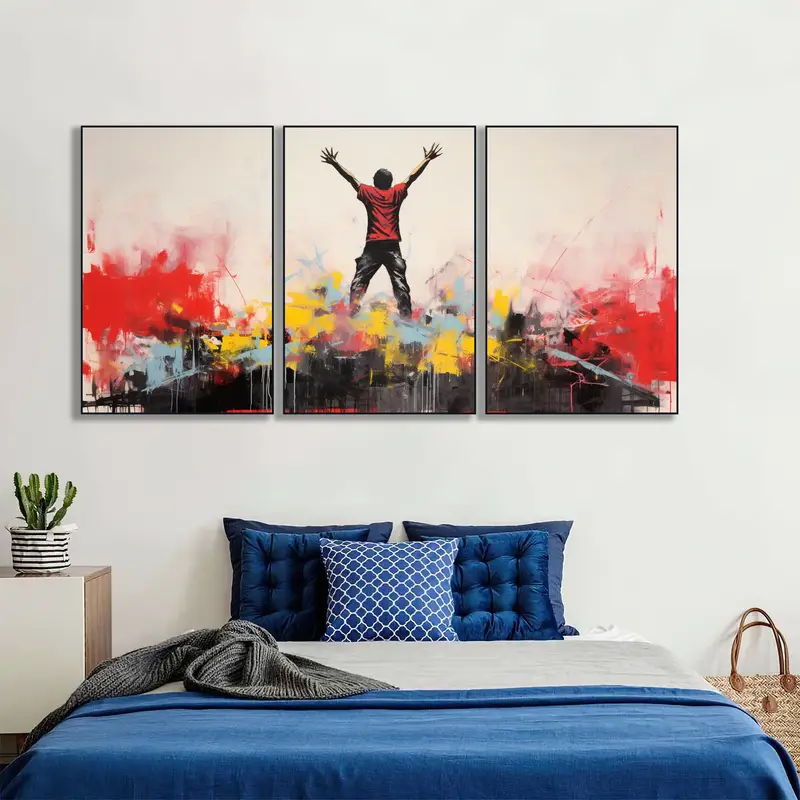The photograph depicts a well-appointed bedroom dominated by a centrally placed bed adorned with a blue comforter, three blue pillows (two dark ones on the sides and a lighter one in the center with a white, grid-like pattern), and a white bed sheet. The backdrop features a white wall with three distinct but coordinated paintings directly above the bed. These artworks, primarily splatter designs with reds, oranges, yellows, blues, and blacks, frame a central piece depicting a man with outstretched arms, dressed in a red shirt and black pants, against a similar color scheme. To the left of the bed stands a white nightstand with a small brown planter housing a green cactus. On the floor to the right, a brown handbag is partially visible, adding a touch of practicality to the scene. Effortlessly combining vivid colors and personal items, the image portrays a comfortable and stylish bedroom space.